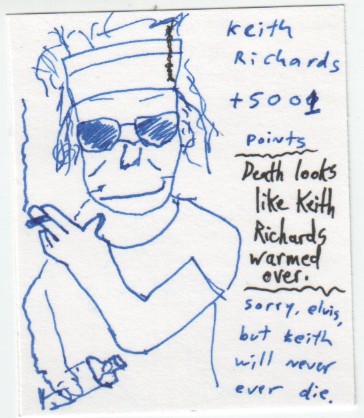This image is a detailed sketch, seemingly drawn on a bar napkin or a small sheet of paper from a notepad. On the left side, it depicts a person resembling Keith Richards, characterized by sunglasses, a bandana tied around their head, and long, scraggly hair. They are wearing a t-shirt. The figure is holding a cigarette with smoke wafting from it in one hand and a liquor bottle in the other. The entire illustration is rendered in blue pen.

On the right side of the image, there is a series of handwritten notes. At the top, in blue text, it reads, "Keith Richards plus 5,001 points." Beneath this, in black ink and separated by squiggly lines, it says, "Death looks like Keith Richards warmed over." Below, in blue text once more, it states, "Sorry, Elvis, but Keith will never, ever die."